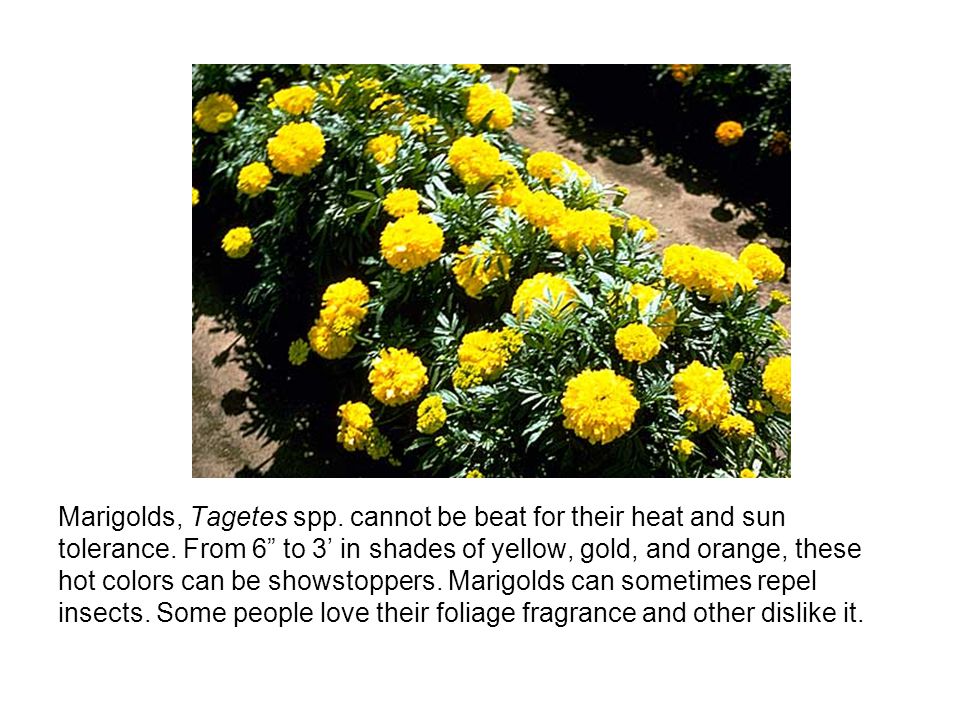The image, taken on a sunny day, shows a vibrant garden scene with a close-up of a large bunch of bright yellow marigold flowers with dark green skinny leaves. They are growing in raised beds, with noticeable furrows in the dirt between the rows. Shadows cast by the flowers are distinct under the bright sunlight, adding depth to the scene. Adjacent to the yellow marigolds, there is a row of orange marigolds, creating a striking contrast. The text below the image reads: "Marigolds, Tagetes spp., cannot be beat for their heat and sun tolerance. From six inches to three feet in shades of yellow, gold, and orange, these hot colors can be showstoppers. Marigolds can sometimes repel insects. Some people love their foliage fragrance, while others dislike it."